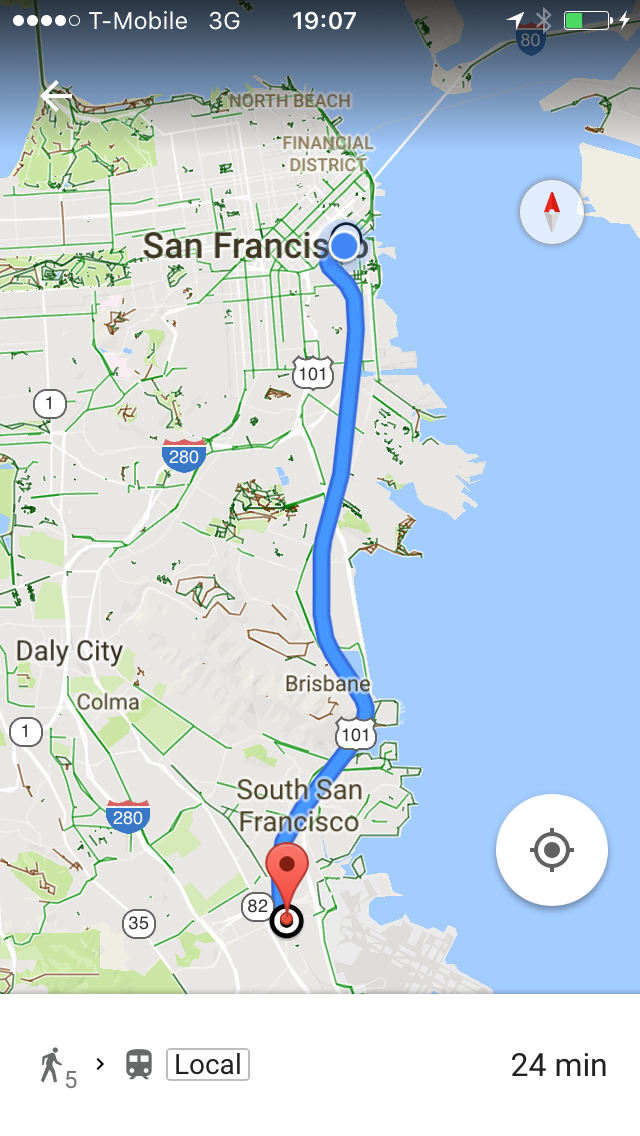**Descriptive Caption:**

The image showcases a screenshot from Google Maps taken on a mobile phone, featuring a detailed view of the San Francisco Bay Area. The map highlights a route from San Francisco to South San Francisco. A blue dot marks San Francisco's location, connected to South San Francisco by a blue and white curvy line representing the travel path. This route traverses the 101 Highway, passing through Brisbane. The final destination in South San Francisco is indicated by a black dot with a white center, paired with a red upside-down teardrop-shaped marker.

Surrounding the highlighted route, the map displays the blue waters of the San Francisco Bay, contrasting with the grayish tones of the densely populated urban areas. Additionally, small green patches denote natural parks scattered throughout the landscape. At the bottom of the image, it notes that the journey begins with a 5-minute walk to a local train station, followed by a 24-minute train ride to reach the destination.